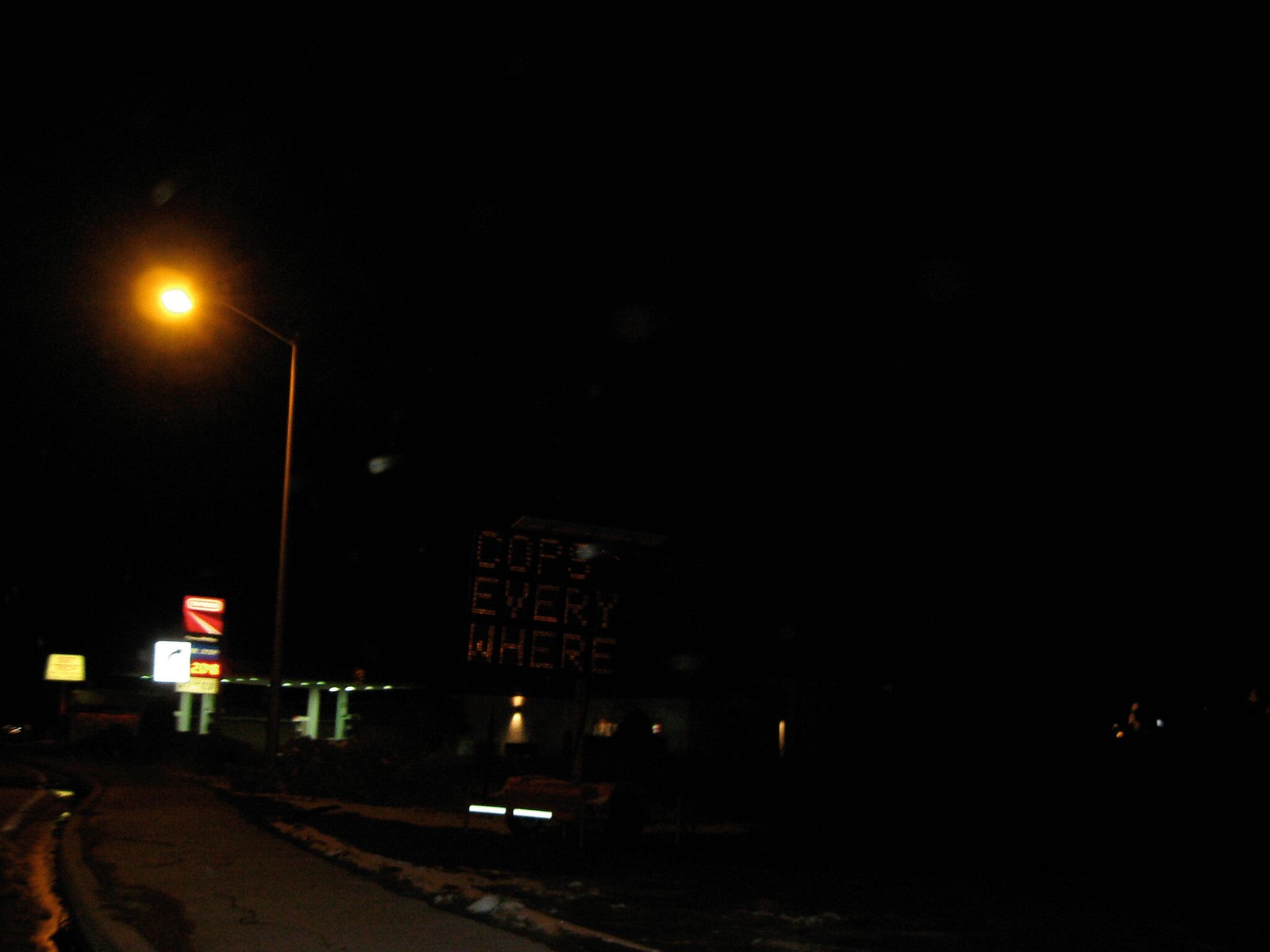This is a nighttime photograph taken with minimal light, making most of the image predominantly dark. A sidewalk curves along the lower left corner, beside which stands a small trailer with a light-up roadside sign displaying the message "COPS EVERYWHERE" in dim orange lettering. Behind and to the left of this sign, a slightly lit-up gas station can be seen, complete with a street sign for gas prices, though the text is too blurry to decipher. The sky and the entire right side of the image are enveloped in darkness, with no visible street lamps. A single streetlight with an amber glow stands in front of the gas station, casting a faint light.